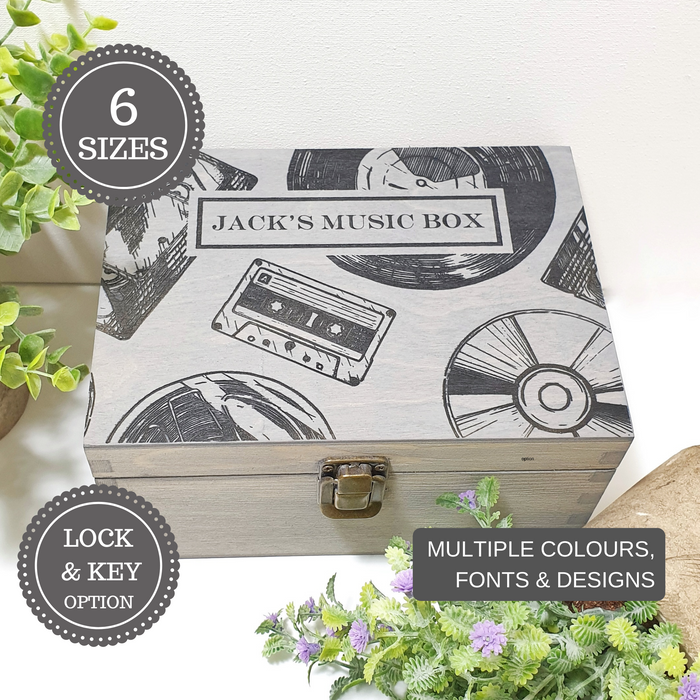The advertisement for Jack's Music Box is set against a creamy white background, featuring the music box centrally placed on a table adorned with two artificial plants. One plant, with light green leaves and purple flowers, is tipped over, adding a touch of casual elegance, while the other, a lighter green flower, stands upright. The music box is a stylish whitewashed gray wooden box with a bronze clasp and prominently displays "Jack's Music Box" on the lid, encircled by black and white images of CDs, vinyl records, and cassette tapes. Various black, perforated circles on the ad communicate key features: the top left circle reads "six sizes," the bottom left indicates "lock and key option," and the bottom right proclaims "multiple colors, fonts, and designs," all in pristine white font. The ad’s layout includes clear corners with vibrant green leaves and purple flowers, enhancing the overall appeal.